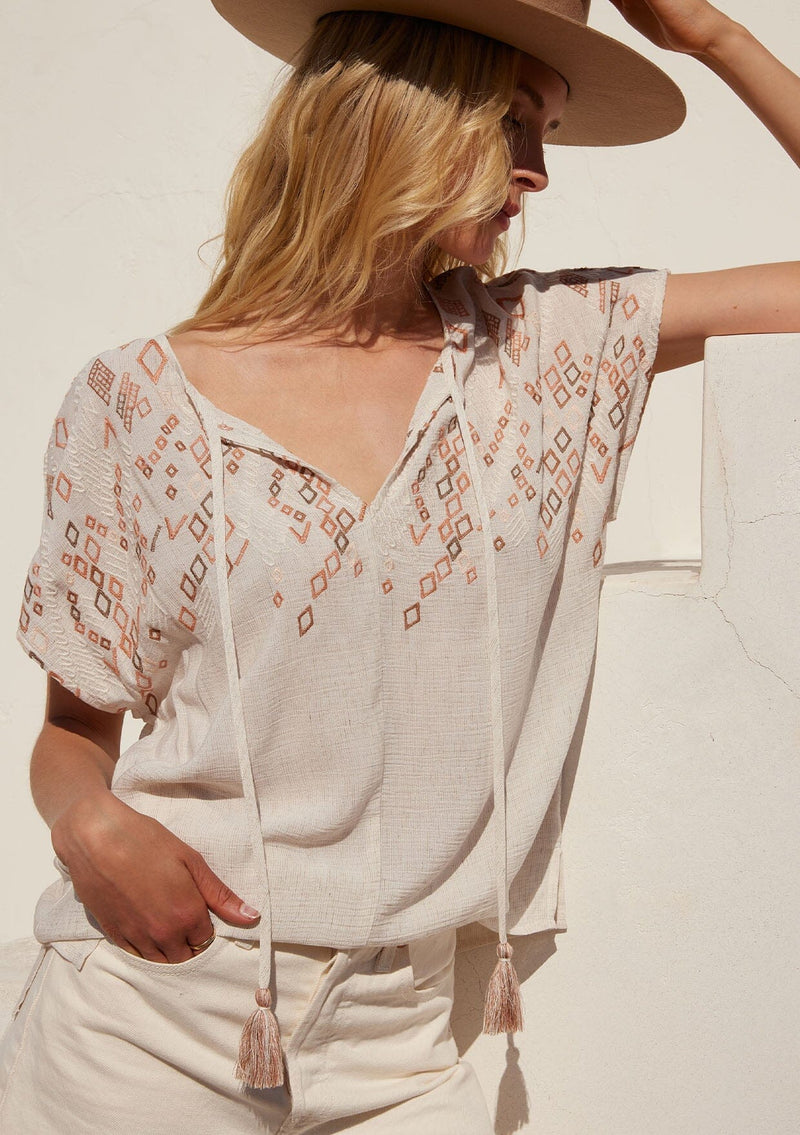In the photograph, a young Caucasian woman with long blonde hair, interspersed with subtle brunette streaks, poses confidently. She dons a cream-colored summery gauze top featuring light brown and pink mauve diamond patterns, giving a rustic yet kawaii appearance. The shirt, loose-fitting and thin, is adorned with decorative tassels dangling from two ties at the neckline, cascading down to her waist. She pairs this top with light cream-colored pants. Enhancing her summery ensemble is a beige straw hat, which she gently touches with her left hand, drawing attention to her stylish accessory. A ring adorns her right forefinger as her hand rests casually in her pocket. The image is artfully cropped at her legs, focusing on her attire and relaxed pose. She stands against a slightly worn white wall with faint cracks and a cutout, adding a textured backdrop to this elegant fashion portrait taken in natural daylight.